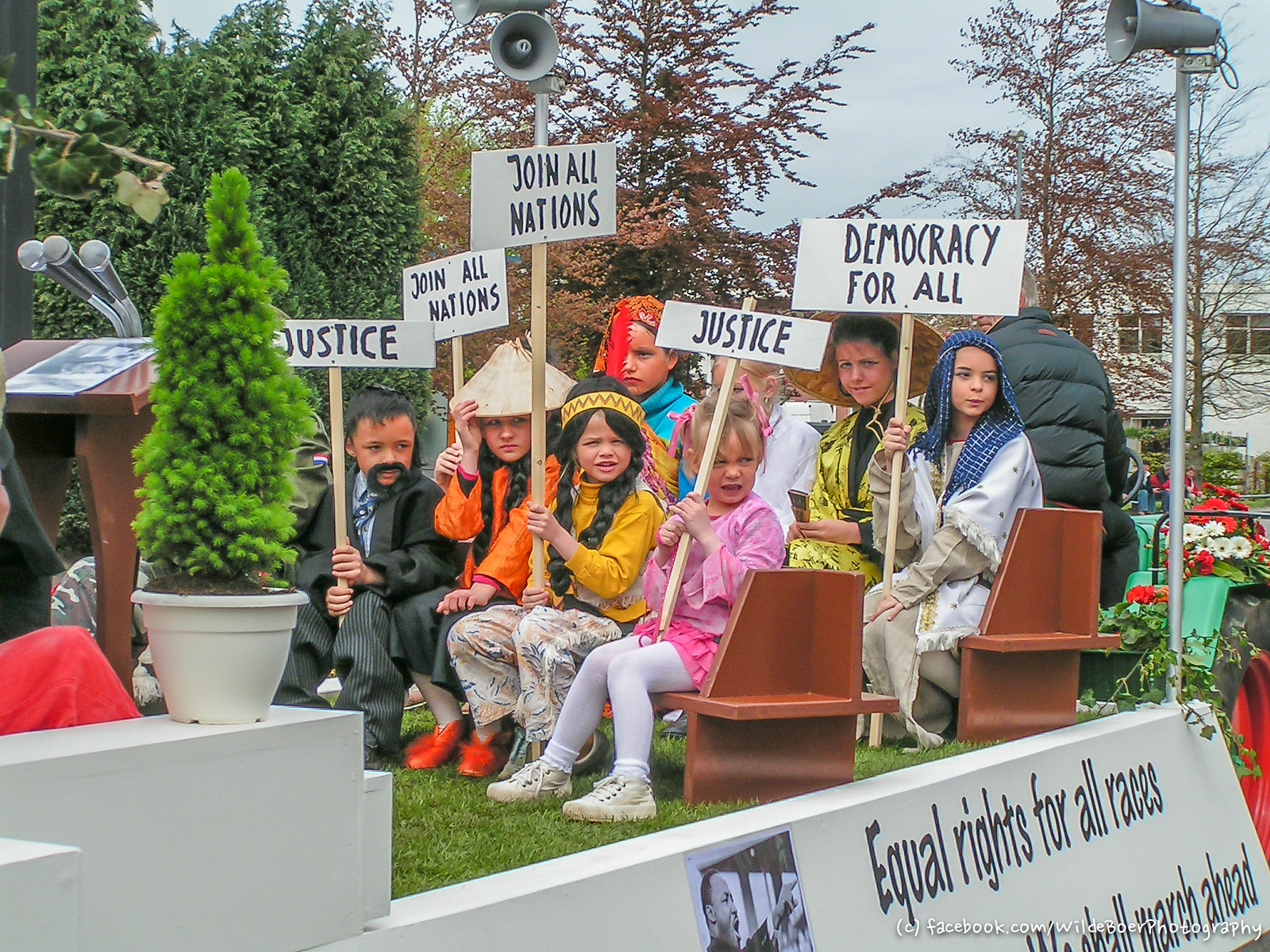In this vibrant outdoor scene, eight children are seated in two rows on benches, each dressed in traditional costumes representing different cultures and holding signs with powerful messages. The children are arranged in front of a backdrop of buildings, trees, and blue skies, amid a peaceful day. They hold white signs with black text; two read "justice," two say "join all nations," and one proclaims "democracy for all." Among the diverse costumes, there's a child dressed in a black suit with a mustache, another in a pink dress with white tights and sneakers, a girl with side braids dressed as an Indian, a child in a triangular hat and yellow Asian attire, and a girl in a white robe with a blue headscarf. Behind them stand large speakers and a man in a black jacket glancing over his shoulder. Notably, a large sign beneath the children reads, "equal rights for all races," featuring an image of Dr. Martin Luther King Jr. and the statement, "we shall march ahead." The arrangement and attire highlight a celebration of cultural diversity and a call for unity and equality.